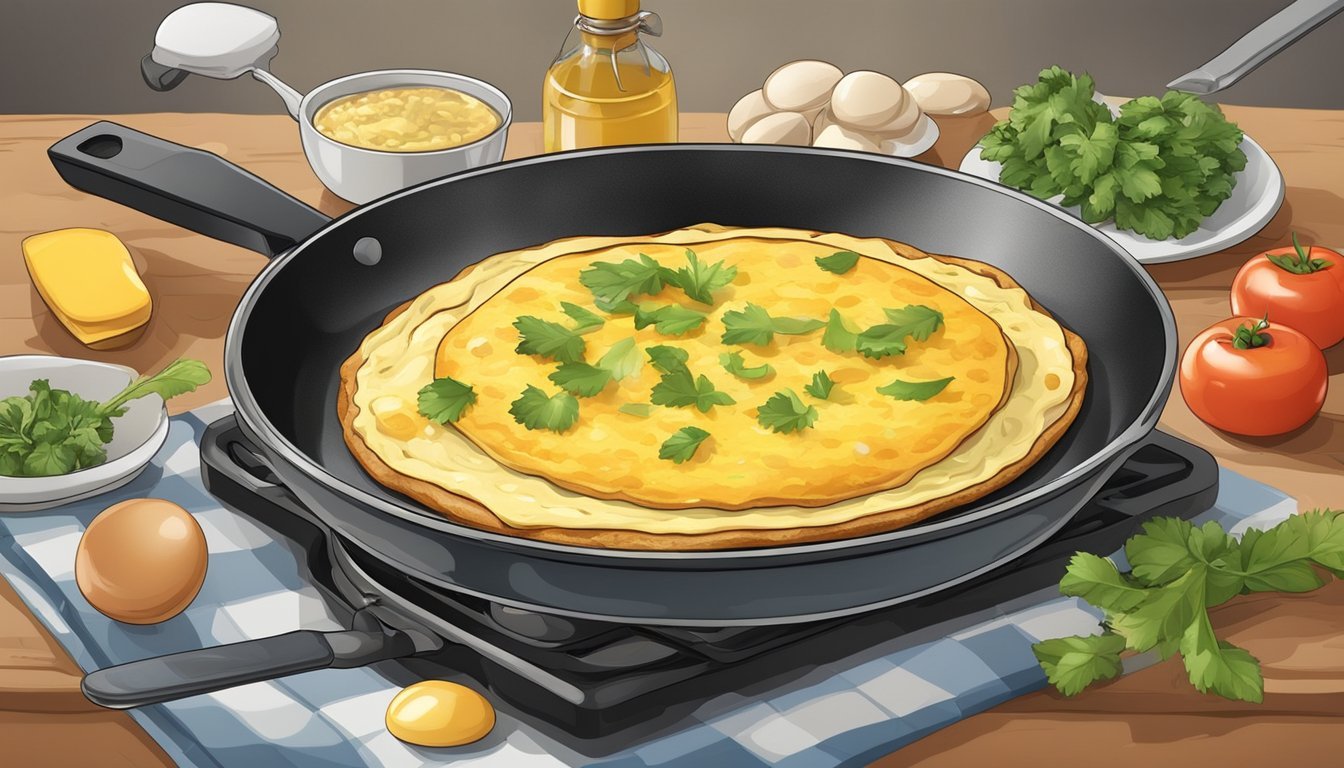This illustration, appearing as if from a cartoon or anime, depicts a breakfast scene set on a brown wooden table that occupies the lower two-thirds of the rectangular image, which measures roughly 5 inches wide by 3 inches high. The backdrop above the table is a light gray wall. Central to the scene is a folded blue and white checkered cloth laying at an angle, serving as the base for a black hot plate. Atop the hot plate sits a matching gray pan containing a yellow omelette garnished with green chives. Surrounding the pan, a variety of breakfast items are meticulously arranged: to the left, there is an uncracked brown egg, a small white bowl filled with more chives, a slab of butter, and a measuring pot with scrambled eggs. Further to the right, there are additional eggshells, a jar of oil at the top center, and a white plate bearing more green garnishes. The right side of the table features two tomatoes and further sprigs of green garnish scattered in the lower right corner, completing this richly detailed, inviting breakfast layout.